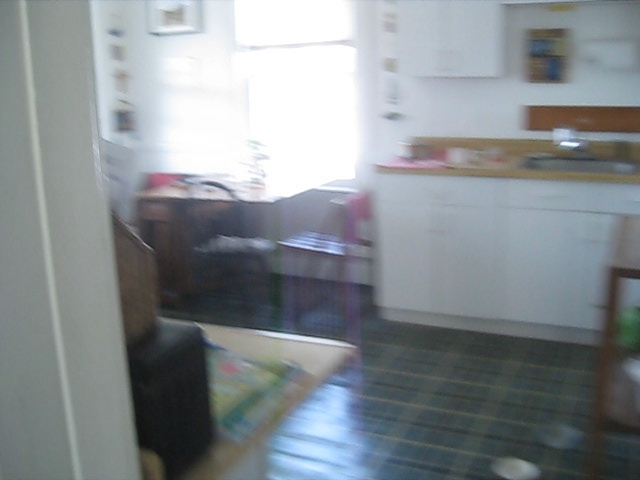The image captures the dynamic scene of a kitchen in motion, with a slight leftward motion blur indicating that the camera was moved quickly to the left. The kitchen interior features a white countertop with a reddish wooden brown counter and matching white cabinets, all set against pristine white walls. The flooring showcases an intriguing green plaid pattern, adding a touch of eccentricity to the space. To the right, a countertop and a tall brown table, likely used for storage, are visible. On the left side, bright sunlight streams through a large window, illuminating the room. Below the window, food bowls are placed on the floor. The wall on the left is adorned with pictures arranged in a vertical stack, adding a personal touch to the kitchen.